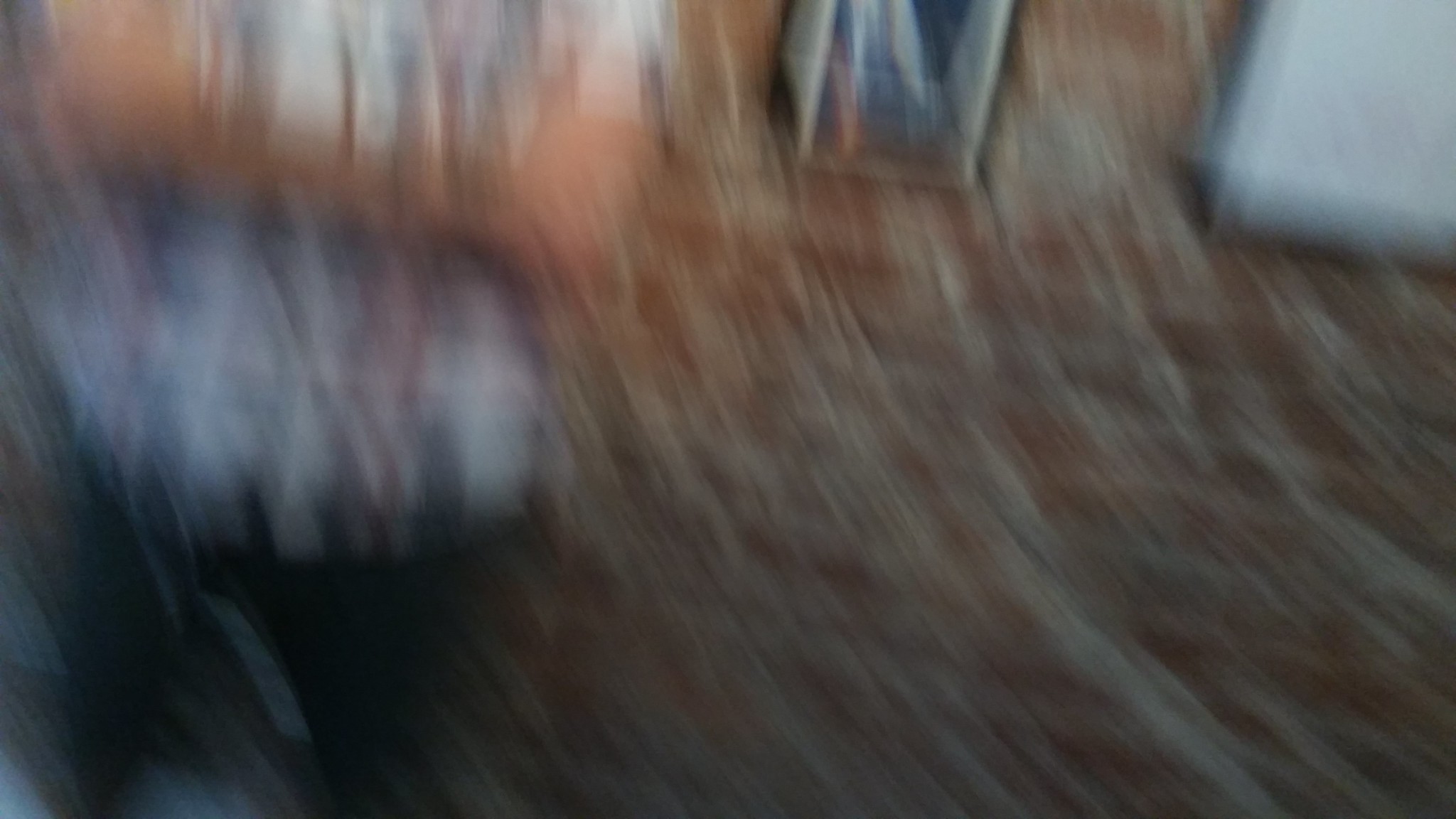A blurred photograph, likely captured while the device was in rapid motion, presents a diagonally slanted perspective. Dominating the image is a distinctive carpet featuring an orangish-red and beige pattern. In the upper right corner, the edge of a wall is faintly visible. The left side reveals the partially captured torso of a person, dressed in a red, white, and blue plaid shirt with arms folded over their stomach. The individual’s head, neck, and area below the knees are cut off by the frame.